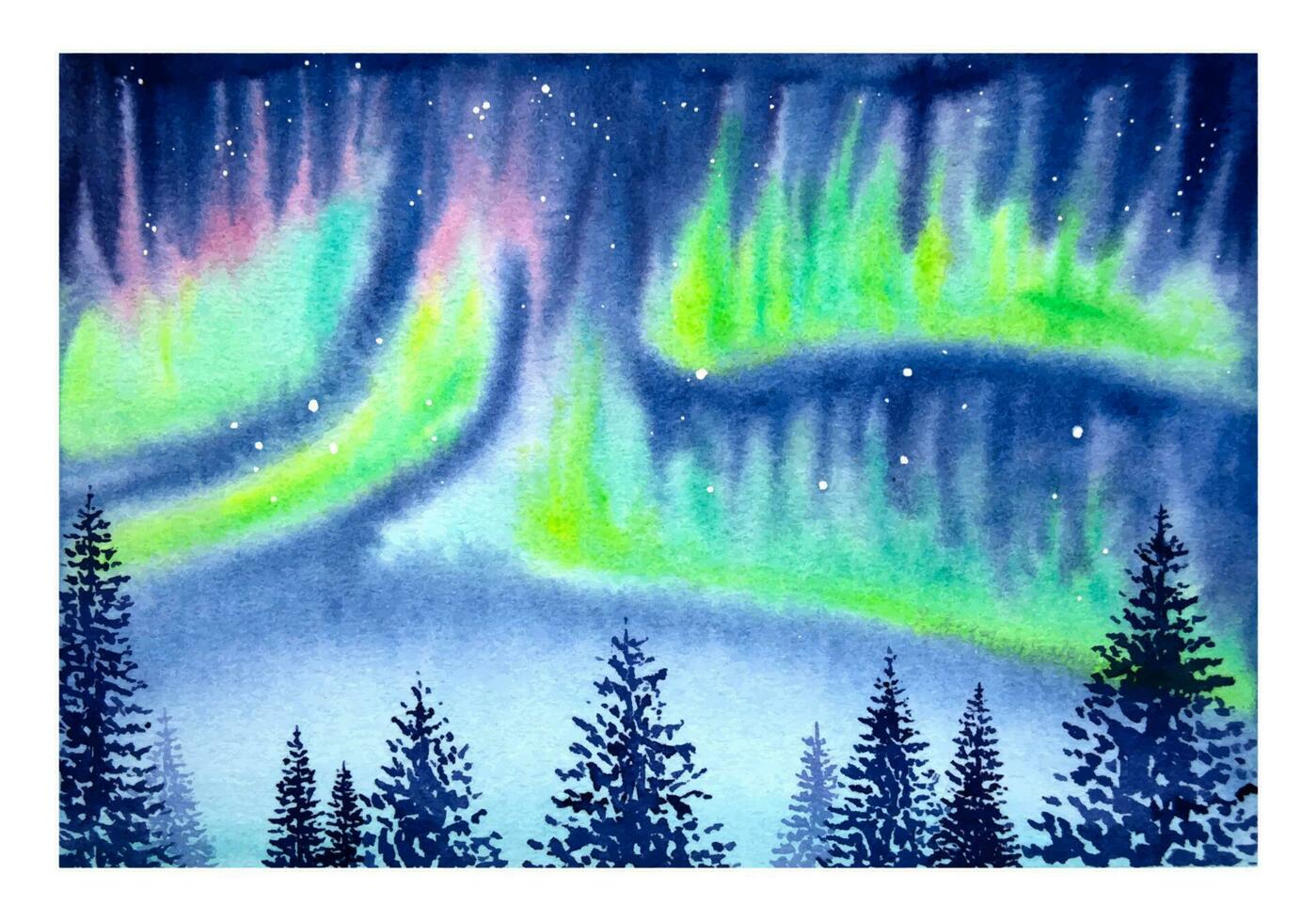This drawing captures a mesmerizing nighttime scene featuring a forest of evergreen, Christmas-type trees at the bottom. Ten dark blue and black conical trees are evenly spread across the soil, with two appearing as faded grayish-blue in the background, adding depth to the forest. The sky, transitioning from a whitish-blue near the horizon to a deep, dark blue at the top, is dotted with white stars. Dominating the sky is a stunning depiction of the Northern Lights, or Aurora Borealis. Broad, amorphous streaks of lime green, yellow, and hints of blue, pink, and red rise up, creating mesmerizing peaks and trails that illuminate the night. The mix of colors and the contrast between the luminous streaks against the darkened sky perfectly evoke the natural splendor of the Aurora Borealis.